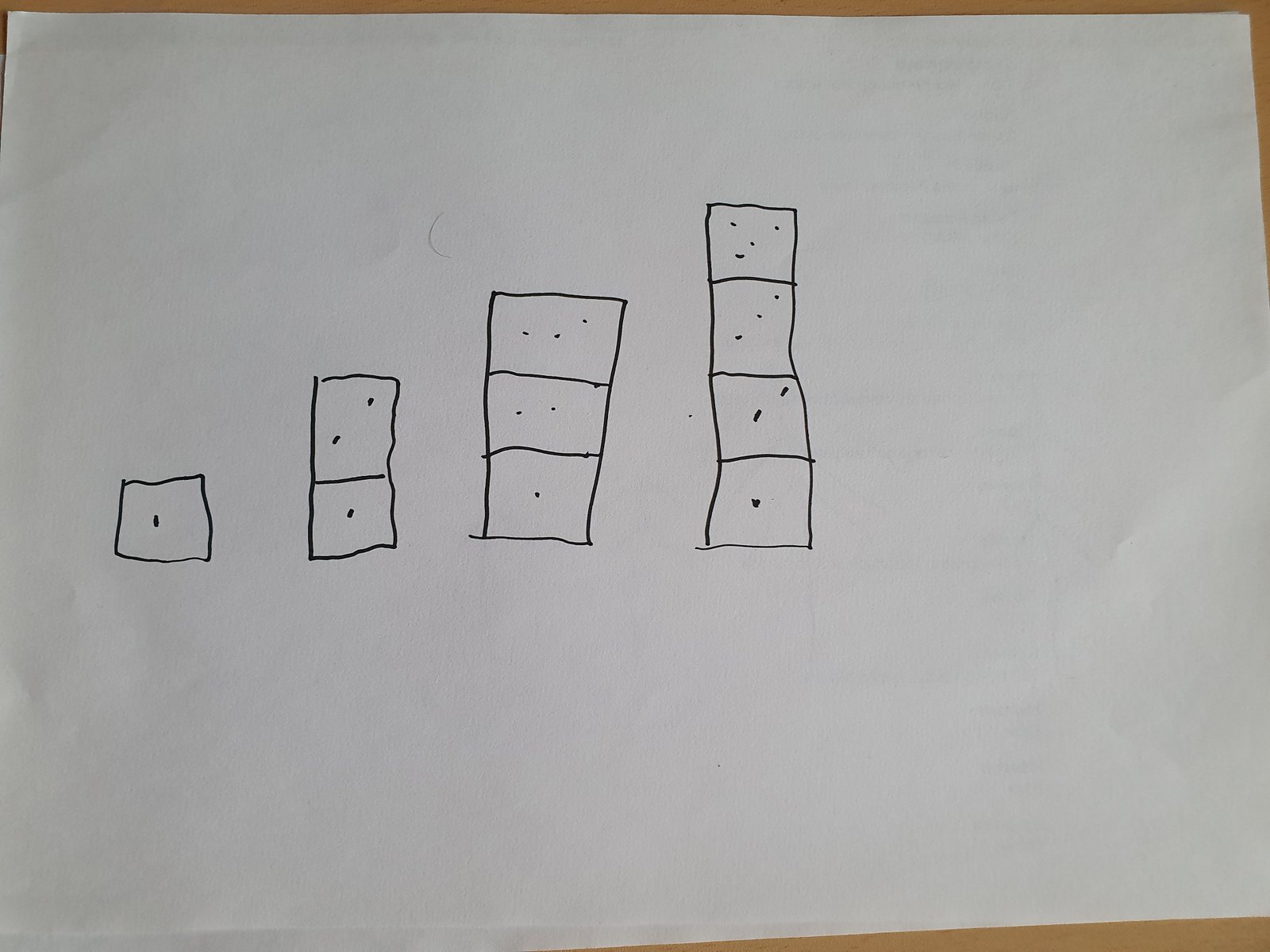This image depicts a detailed hand-drawn pattern on a white sheet of paper, resting on what appears to be a medium-brown wooden table, visible along the top and bottom right edges of the frame. The drawing features a sequential arrangement of small squares, each containing black dots. 

Starting from the left-hand side of the paper, there's a small square with a single black dot. Moving rightward, the next square again has one black dot, but is overlaid with a second square featuring two black dots. Continuing this pattern, another square with one black dot is topped by a second square with two black dots, followed by a third square containing three black dots. Progressing further to the right, the sequence becomes more complex: a square with one black dot is beneath a second with two black dots, a third with three black dots, and finally, a fourth with four black dots. 

In the middle right-hand corner of the paper, a noticeable crease or fold mark suggests the paper was previously folded and has since been flattened out. The meticulous arrangement of squares and dots creates a fascinatingly structured visual that stands out against the pristine white backdrop.